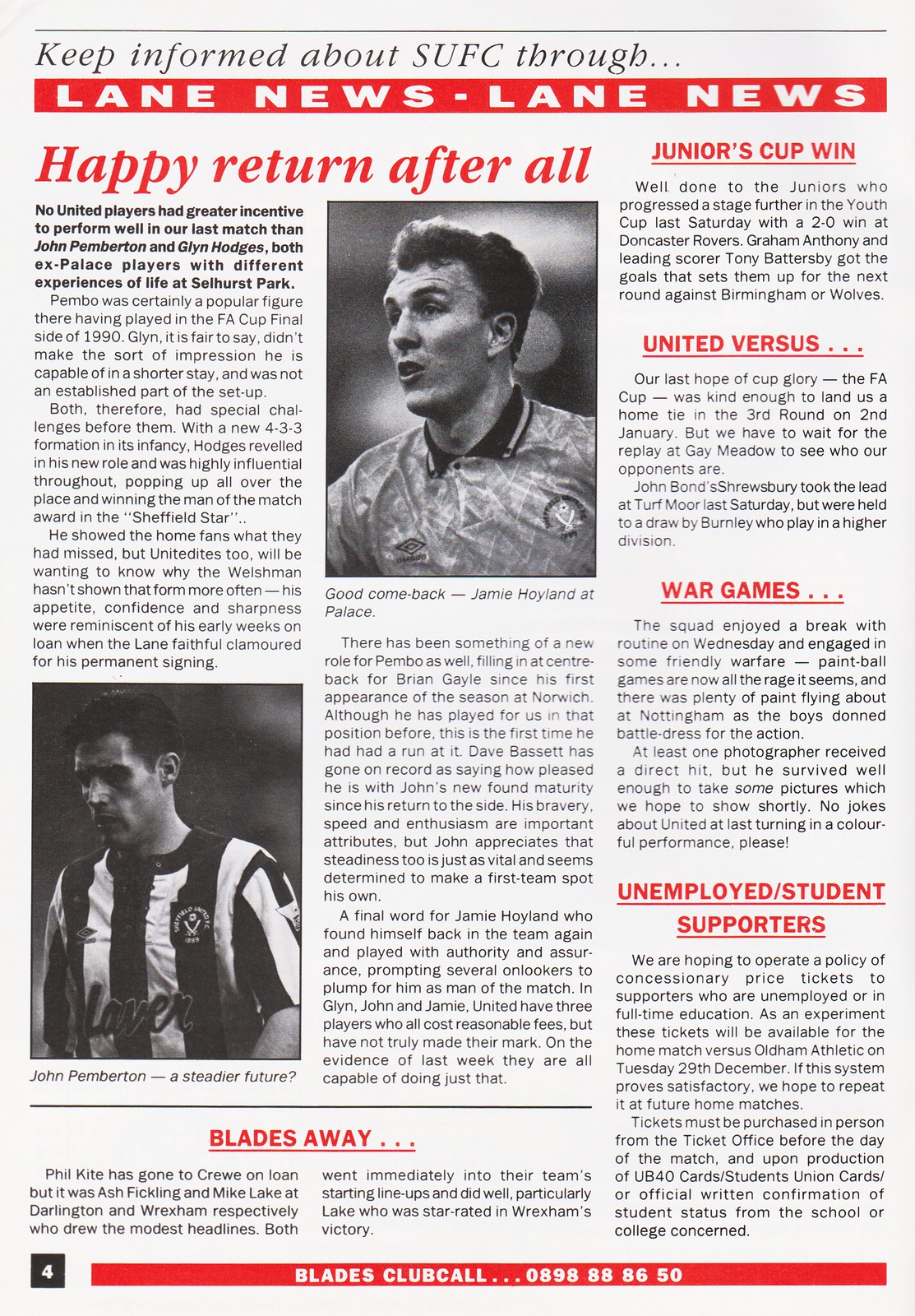The image appears to be a vivid and clearly legible page from a magazine or newspaper, emphasizing news about SUFC through Lane News. At the top, a prominent red banner reads "Keep informed about SUFC through Lane News, Lane News." The main article, titled "Happy Return After All," spans the first two columns on the left, featuring detailed text below two photographs. One photo, located at the bottom of the left column, appears to be of soccer player John Pemberton, while another photo in the middle column shows Jamie Hoyland at Palace.

On the far right column, several smaller news excerpts are listed, starting with “Junior's Cup Win,” followed by “United versus,” “War Games,” and “Unemployed/Student Supporters.” Additionally, the phrase "Blades Away" is prominently displayed, spanning the bottom of the first two columns in red text. At the very bottom, another red banner reads "Blades Club Call," accompanied by a potential phone number: 0898 8888650. The page, numbered four, offers a comprehensive and visually engaging presentation on SUFC-related news.